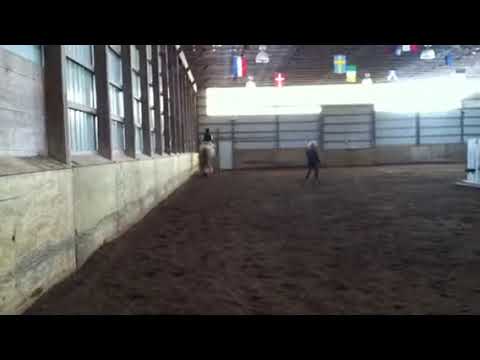The image depicts an indoor horse training facility characterized by a vast dark brown dirt arena. Central to the scene is a white horse with a black tail, facing the back wall, ridden by a person in a black suit. To the right of the horse, a second individual dressed in dark clothing walks across the dirt. The background features a mixed-material wall, with a lower brown section, topped by wooden planks framed with gray bars. Above the wall, flags from various countries hang from the rafters, including a blue, yellow, and red flag, a red flag with a white cross, a blue flag with a yellow cross, and a green, white, and orange-striped flag. The roof structure, supported by brown metal columns, also holds several lights. Overall, the lighting suggests daylight filtering in, likely through overexposed cutouts or windows, creating a partially bright and muted visual atmosphere.